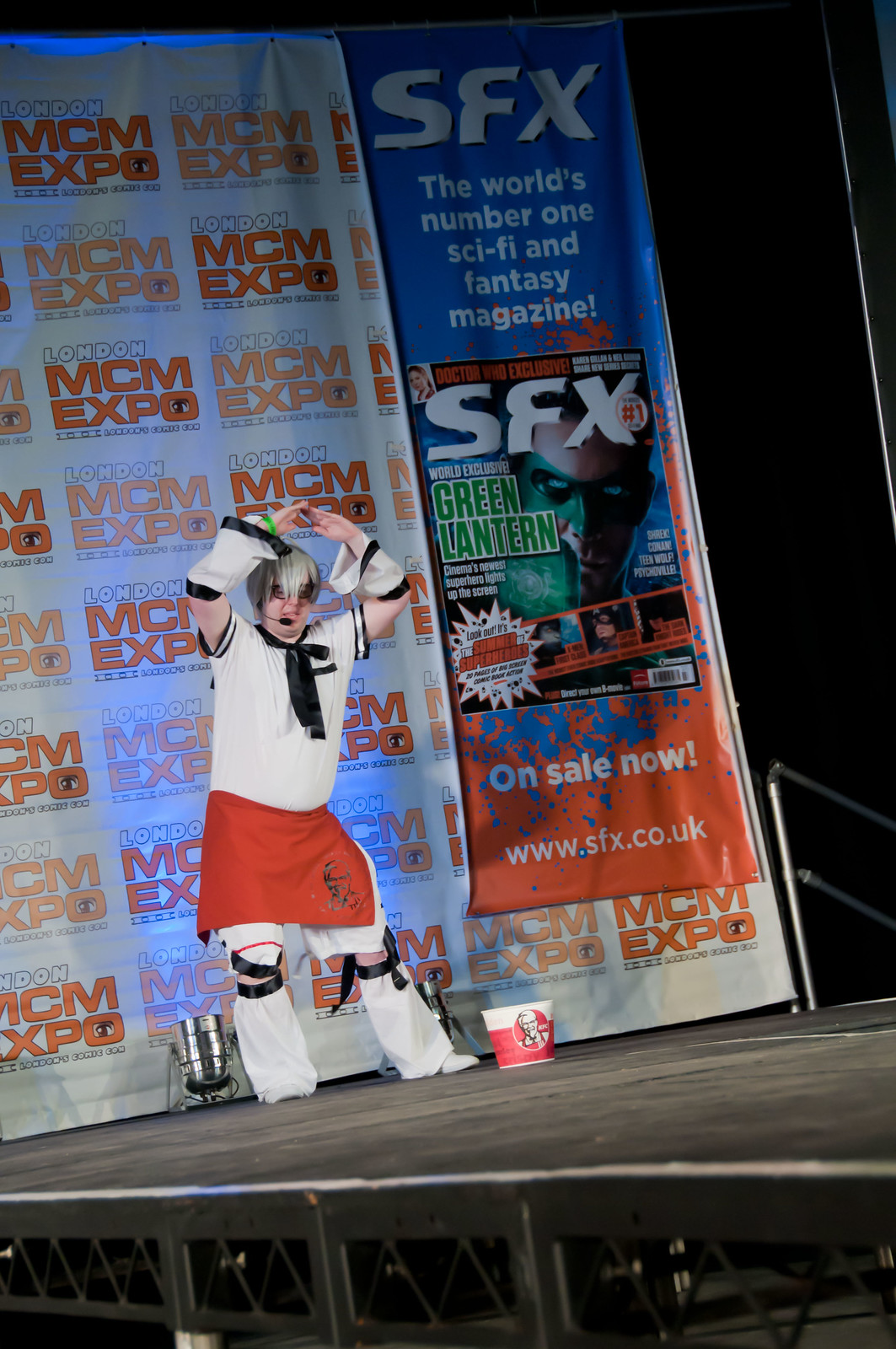A detailed photograph captures a person performing on a slightly askew stage at the London MCM Expo. The backdrop prominently features a large sign that reads 'London MCM Expo' alongside an expansive banner for SFX, labeled as "the world's number one sci-fi and fantasy magazine." Displayed on the banner is an issue of SFX magazine with the Green Lantern on the cover and an inscription that reads "On sale now www.sfx.co.uk." The person on stage is striking a pose with their arms raised above their head, touching at the fingertips, resembling a roof shape. They are dressed in a distinctive outfit: a white short-sleeved shirt adorned with black details, matching white shorts, and a red apron extending from their waist to just above their knees. Their lower legs are covered with something akin to leg warmers, and their spiky hair, styled in shades of yellow and gray, gives them a standout look. At their feet, a bucket of Kentucky Fried Chicken is clearly visible, distinct with its red and white design featuring the Colonel Sanders logo. The stage itself is black, and a few lights illuminate the base of the backdrop, casting a spotlight effect that draws attention to the performer.